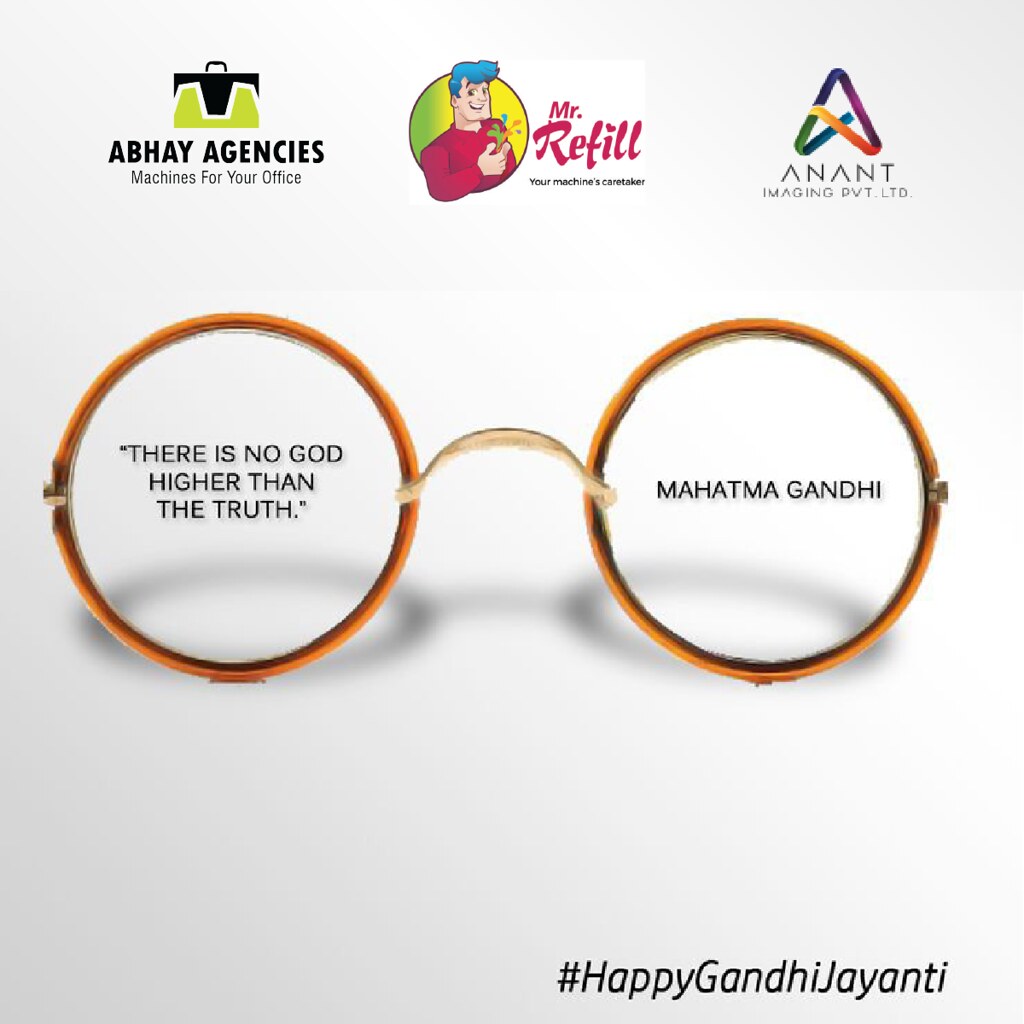The image appears to be an advertisement on a white background. In the top left corner, there's a bag that is green and black, accompanied by text in all capital letters reading "ABHAY AGENCIES." Below this, it states, "Small Print Machines for your office." To the right of this is a logo of a man with blue hair wearing a red shirt with the text "Mr. Refill - Your machines caretaker." Further to the right is another logo with "ANANT" at the bottom, followed by "Imaging Imaging Pvt. Limited." The central part of the image prominently features a large pair of wire-framed round glasses, which lack visible arms. Inside the left lens of the glasses, there's a quote in black text that reads, "There is no God higher than the truth," attributed to Mahatma Gandhi, whose name appears in the right lens. The bottom right corner of the image displays the hashtag "#HappyGandhiJayanti."